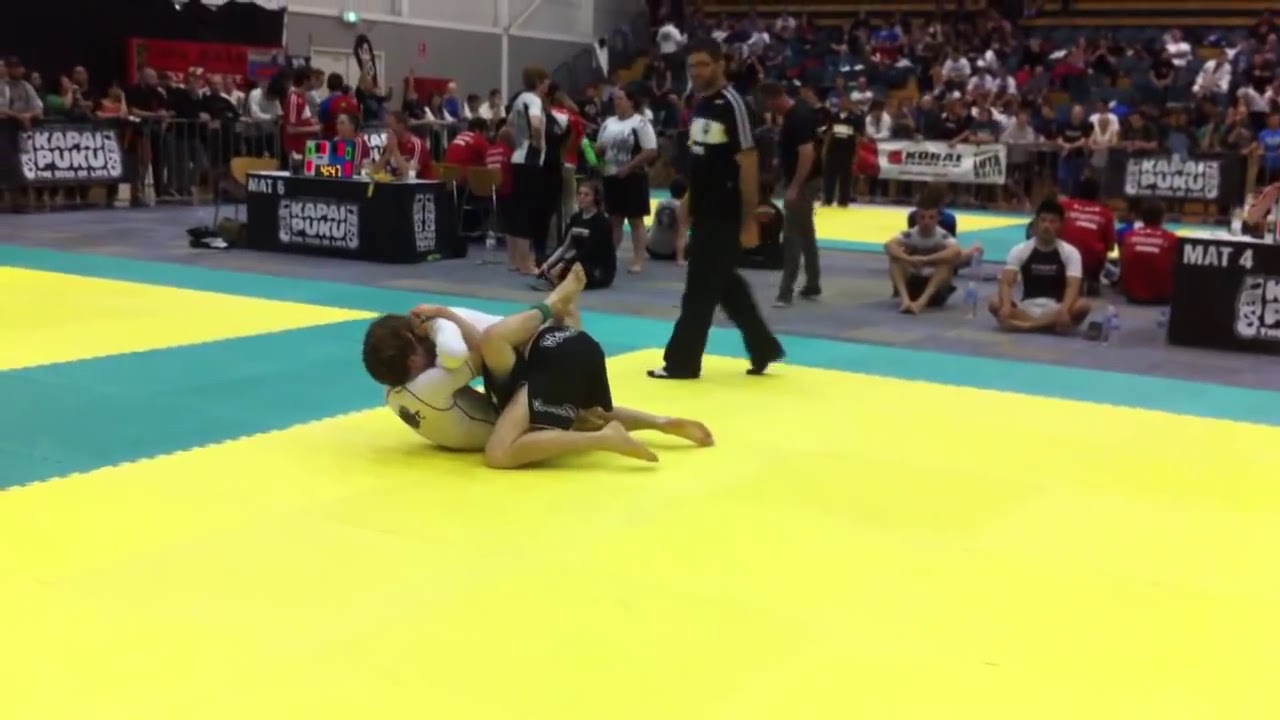The image captures the intensity of a wrestling match taking place in a brightly lit gymnasium, with rows of seats and bleachers filled with spectators in the background. At the center of the action, two young male wrestlers are engaged on a mat that has a bright yellow center with green borders. The gym has a total of four such yellow square mats—two in the foreground and two in the distance. A referee dressed in black pants and a black shirt with white stripes down the arms monitors the match closely. The wrestler on the bottom has a strong hold around his opponent's neck and upper arms, with his legs locked around the opponent's waist, while the other wrestler is on his knees, struggling to gain control.

In the middle of the mats are two black tables with banners that have white, rounded letters spelling out "K-A-P-A-I-P-U-K-U," possibly indicating the name of the organization or teams involved, and labeling the mats as "mat six" and "mat four." Alongside the mats, other young wrestlers, possibly waiting for their turn, sit watching the match unfold. Spectators are separated from the competitors by a metal gate, creating a clear division between the action and the audience. There are individuals wearing red t-shirts among the spectators, contributing to the vibrant and busy atmosphere of the event.